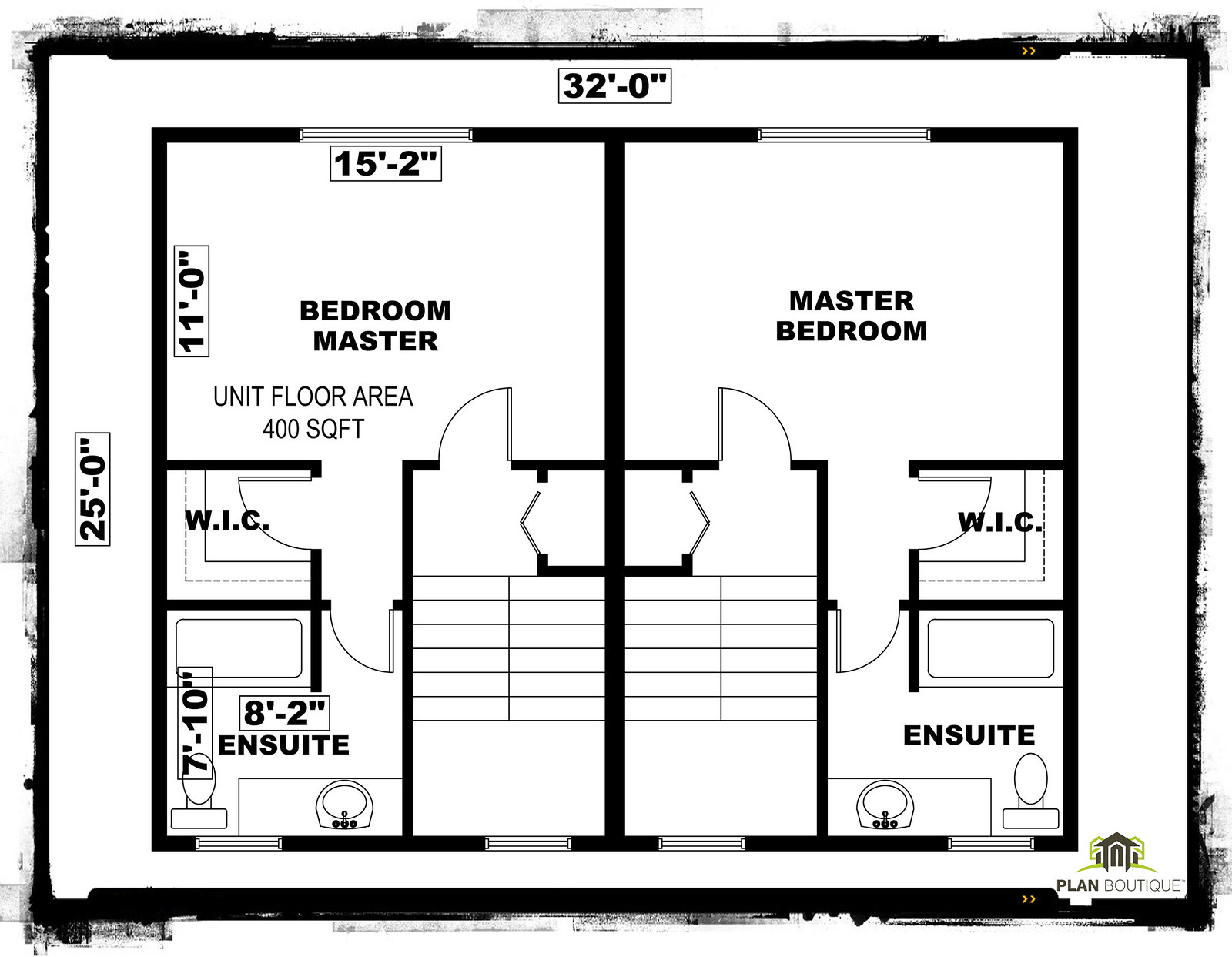This architectural drawing depicts a detailed floor plan of a house viewed from above, outlined with thick black lines representing the walls and perimeter. The structure includes an encompassing walkway or porch. The overall dimensions of the house are stated as 25 feet 0 inches vertically and 32 feet 0 inches horizontally.

Inside, there is a master bedroom unit with a specified floor area of 400 square feet. The dimensions of this inner space are 11 feet 0 inches vertically and 15 feet 2 inches horizontally. Located in the middle of the top wall of this room is a window.

Adjacent to the right of this master bedroom is another master bedroom, which also features a window at the top wall but lacks specified dimensions. Besides this bedroom, there is a WIC (walk-in closet) and an en-suite bathroom. The en-suite bathroom on the left corner measures 7 feet 10 inches by 8 feet 2 inches and includes a sink, toilet, and bathtub. Similar features are present in the en-suite bathroom on the right-hand corner.

Each bedroom has corresponding walk-in closets, and there is a staircase providing access to other floors, along with open doors leading into these bedrooms. The precise arrangement and features of these spaces illustrate a well-thought-out design within the overall architectural blueprint.